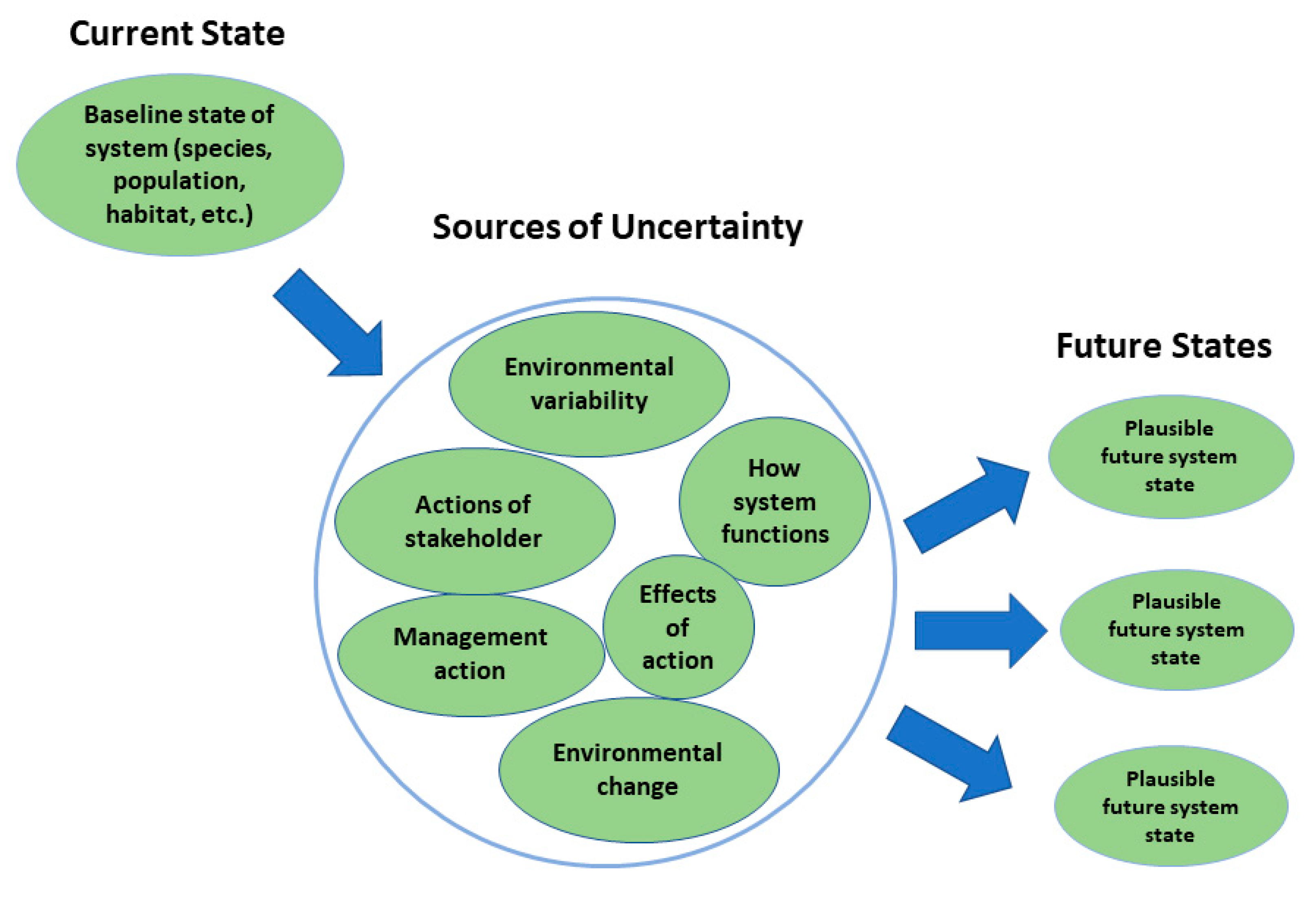This is a detailed infographic flowchart set against a white background. In the upper left, there’s a green oblong bubble labeled "current state" with the black text inside reading "baseline state of system, species, population, habitat, etc." A blue arrow points from this bubble to a large central bubble outlined in blue with a white background labeled "sources of uncertainty." Within this central bubble, there are several green bubbles outlined in blue with black text, detailing various factors such as "environmental variability," "how system functions," "effects of action," "environmental change," "management action," and "actions of stakeholder." From this central bubble, three darker blue arrows branch out to three smaller green bubbles, each labeled "future states." Inside each of these smaller bubbles is the text "plausible future system state."